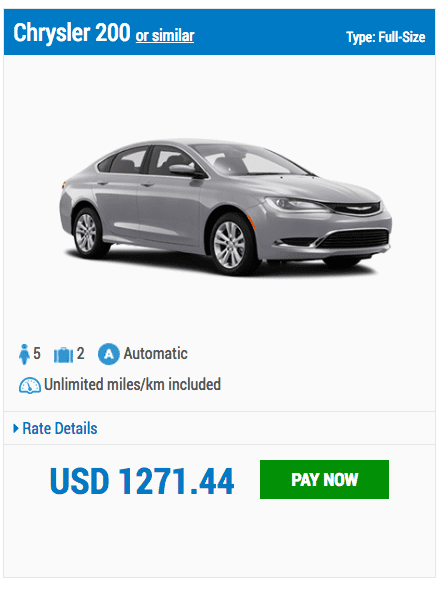**Chrysler 200 or Similar – Full Size Car Rental Ad**

The advertisement showcases a simple yet informative layout featuring a Chrysler 200 or a similar full-size car. The main title is set against a blue background with bold white text that reads "Chrysler 200 or similar," with "or similar" underlined for emphasis. To the right of the title, the text specifies the type as "Full Size."

A clean product photo of a silver-colored, four-door sedan is prominently displayed over a white or transparent background, enhanced with a subtle drop shadow beneath the car. The image conveys a sleek design and practical functionality.

The car's capacity is highlighted with icons indicating it can accommodate up to five people, alongside a briefcase icon suggesting space for two pieces of luggage. An intuitive blue circle with an 'A' denotes that the car has an automatic transmission. Additionally, a speedometer icon indicates that unlimited miles or kilometers are included with this rental package.

The detailed rate information is prominently displayed as "USD $1,271.44", and a green button with white text invites users to "Click to Pay Now," providing a clear call to action. This ad likely represents a listing from a car rental service or booking app, offering a straightforward and user-friendly interface for potential customers.